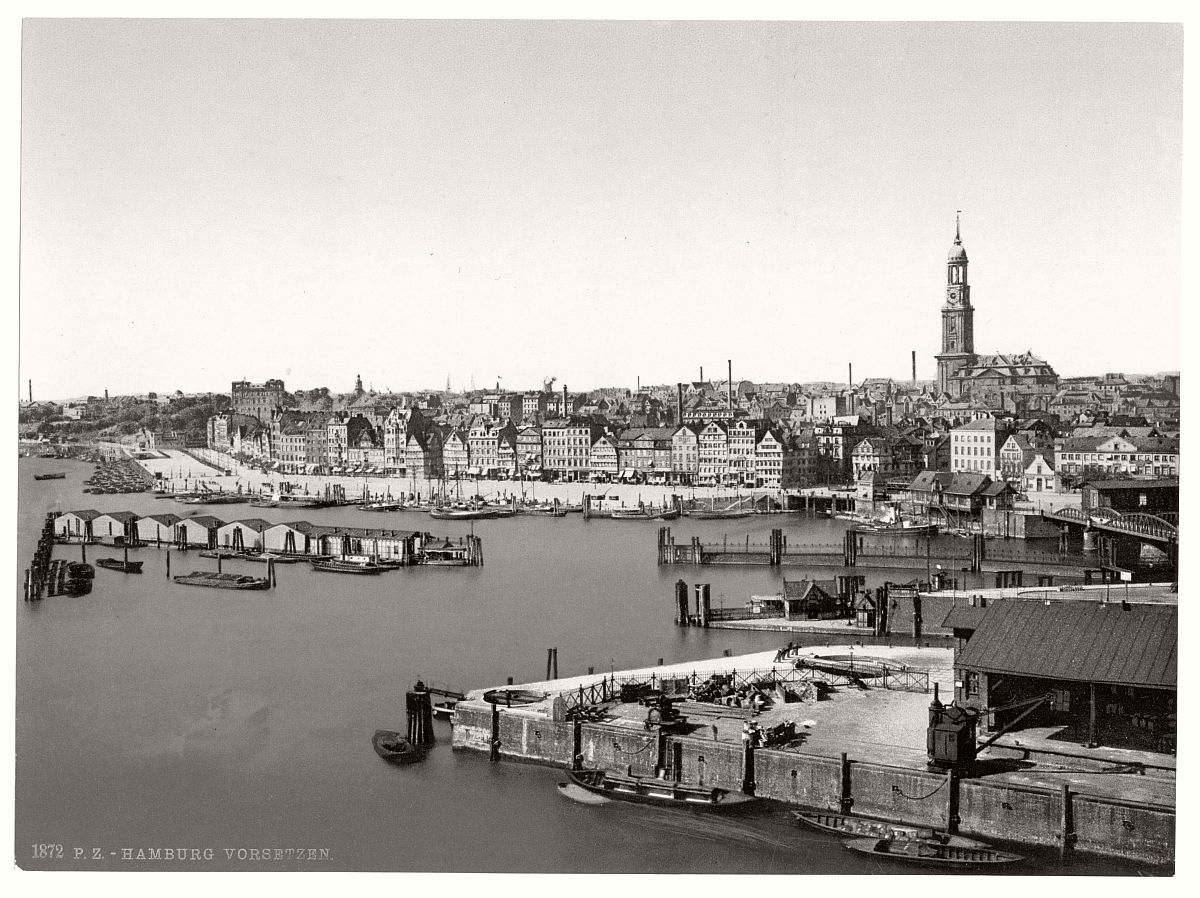This black-and-white photograph, possibly an old postcard from 1872, illustrates the waterfront of Hamburg, Germany, with the caption "1872 P.Z. Hamburg Vorbitzen" inscribed at the bottom. The high-quality image captures a bustling nautical scene in daylight, showcasing remarkable detail given its 150-year age. In the foreground, the docks and shipyard with dry docks are clearly visible, featuring steamboats and floating structures resembling small huts. The wide expanse of water, likely an ocean or broad river, separates the viewer from the cityscape on the opposite shore. The skyline is dominated by multi-story 19th-century European buildings, characterized by triangular gable roofs and industrial smoke pipes. Among these structures stands a prominent church with a towering bell steeple and another significant building that might be a city hall or courthouse, distinguished by its seven or eight stories. A bridge is visible to the right, further enhancing the intricate urban tableau. The photograph, devoid of people except for a single individual, meticulously focuses on the architectural and industrial elements of this historical port city.